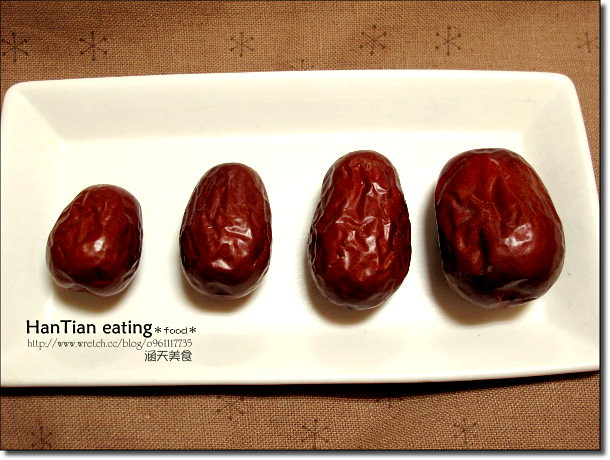A photograph features a long, off-white rectangular dish resting on a brown, burlap-like cloth that is adorned with alternating darker tan snowflakes. The dish holds four dark red, wrinkled fruits, which are likely dates based on their prune-like skin and varying sizes. Arranged horizontally from left to right, the leftmost fruit is the smallest and rounded, the next is egg-shaped, the third is longer with the most wrinkles, and the rightmost is the largest and roundest. In the bottom left corner of the dish, text has been added digitally, reading "Han Tian Eating *food* http://www.retch.ee/blog" in black letters. Below this, some Chinese characters are also visible.